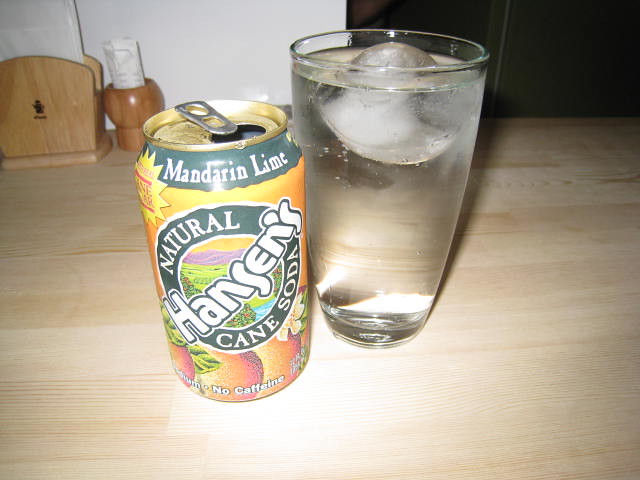A close-up photo captures a tantalizing scene centered around a can of soda. Resting on a light-colored brown table with prominent horizontal wood grain, the can of Hansen's Mandarin Lime Cane Soda stands out. The pull tab is lifted, signaling the can has been opened, and inviting the observer to a sensory experience. The can is vibrant, sporting a colorful design with a backdrop of medium blue and white lettering. The golden and orange hues of the can are complemented by the illustrated fruits at the bottom, resembling oranges, giving a nod to its refreshing mandarin lime flavor. In the foreground, a clear glass with simple, elegant sides is filled to the brim with the bubbly soda, crowned by a single large chunk of ice. The scene captures a refreshing moment, perfect for a hot day. In the background, a light tan napkin holder with white napkins and another brown holder with unspecified items add a touch of everyday realism to this inviting tableau.